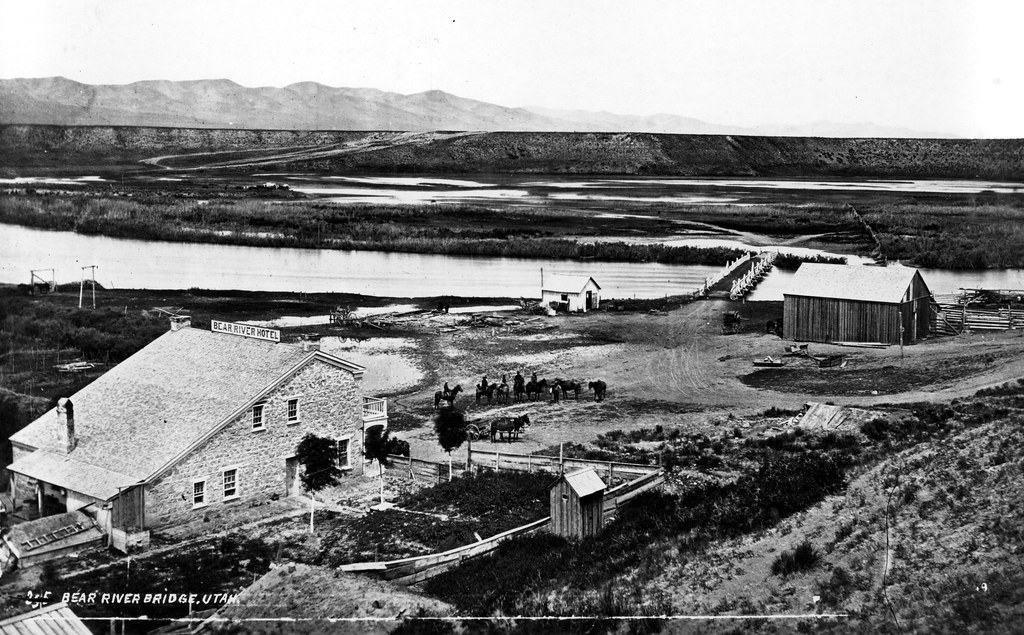This black-and-white photograph, likely taken in the mid-1800s, depicts a sparse, Old West-style scene adjacent to a body of water that runs horizontally through the image. In the foreground, clusters of people and cowboys, both on horseback and on foot, populate the dirt ground. Prominent in the photograph are the Bear River Hotel and a large wooden barn, the former featuring a sign atop its roof that clearly reads "Bear River Hotel." To the right of the hotel, there's a smaller, darker building with a peaked roof, and nearer to the water, a very small white shed or house with a similar roof design. A bridge spans the river in the background, with a mountain range featuring distinct peaks visible further back. Notably, at the bottom left corner, the photograph is labeled in all capital white letters: "Bear River Bridge, Utah."